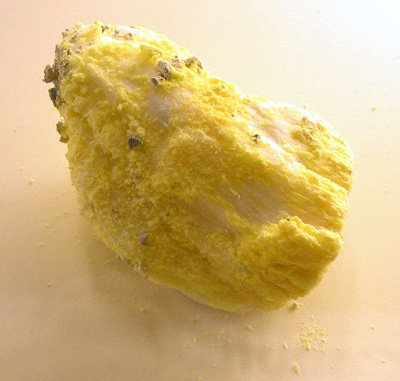A close-up image captures a large, yellow object that takes up about 80% of the frame, situated directly in the center on a plain, off-white surface. The figure, possibly a dried-out lemon but also speculated to be a rock with yellow sediment, exhibits a crumbly and flaking exterior with small yellow fragments broken off. The object has brown spots on the top left and small green patches signaling the start of mold. There is natural or artificial light illuminating the top right of the object, suggesting an indoor setting, potentially a kitchen or a room with a window. The surface underneath the yellow layer reveals a peach to white underbelly, adding to the ambiguity of its true nature.